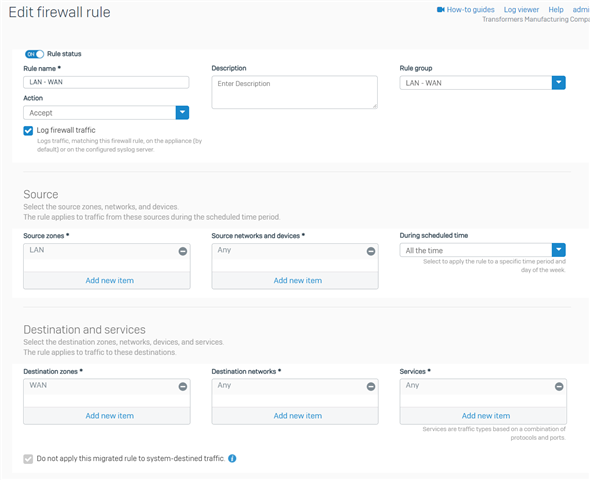Here is a detailed and cleaned-up caption for the image described:

---

In the top left corner of the image, the heading "Edit Firewall Rule" is displayed. On the right side of the screen, there is a light blue icon representing a video, with the label "How-to Guides" next to it. Below these elements, the menu items "Log Viewer" and "Help" are listed, followed by "Add Me." 

Underneath the title "Transformers Manufacturing - Correct," there is a large white box. This box is titled "World Status," with a subheading of "World Name" and an empty input field labeled "lan-wan." 

Directly below this, there is a section labeled "Action," where the option "Accept" is selected. Within this section, a checked box indicates that "Log Firewall Traffic" is enabled, specifically stating, "Logs traffic matching that firewall rule on the appliance (by default) are on the configured syslog server."

Towards the middle of the page, there is a section labeled "Description," an empty field with the placeholder text "Enter description." To the right of this, the label "Rule Group" is present with the option "lan-wan" selected.

A horizontal line divides this area from another large white box below it. In this section, the label "Source" directs users to select the source zones, networks, and devices that the rule applies to during the scheduled time period. 

This section contains three columns:
1. The first column "Source Zones" features entries "LAN" and "New Item."
2. The second column "Source Networks and Devices" shows the options "Any" and "New Item."
3. The third column "During Scheduled Time" has the option "All the time," with details to "select to apply the rule to a specific time period and day of the week."

Another horizontal line is present before the final white box, which is labeled "Destination Services." This box instructs users to select the destination zones, networks, devices, and services to which the rule applies.

This final section is divided into three columns:
1. The first column "Destination Zones" lists an entry labeled "WAN."
2. The second column "Destination Networks" has the option "Any."
3. The third column "Services" contains the option "Any."